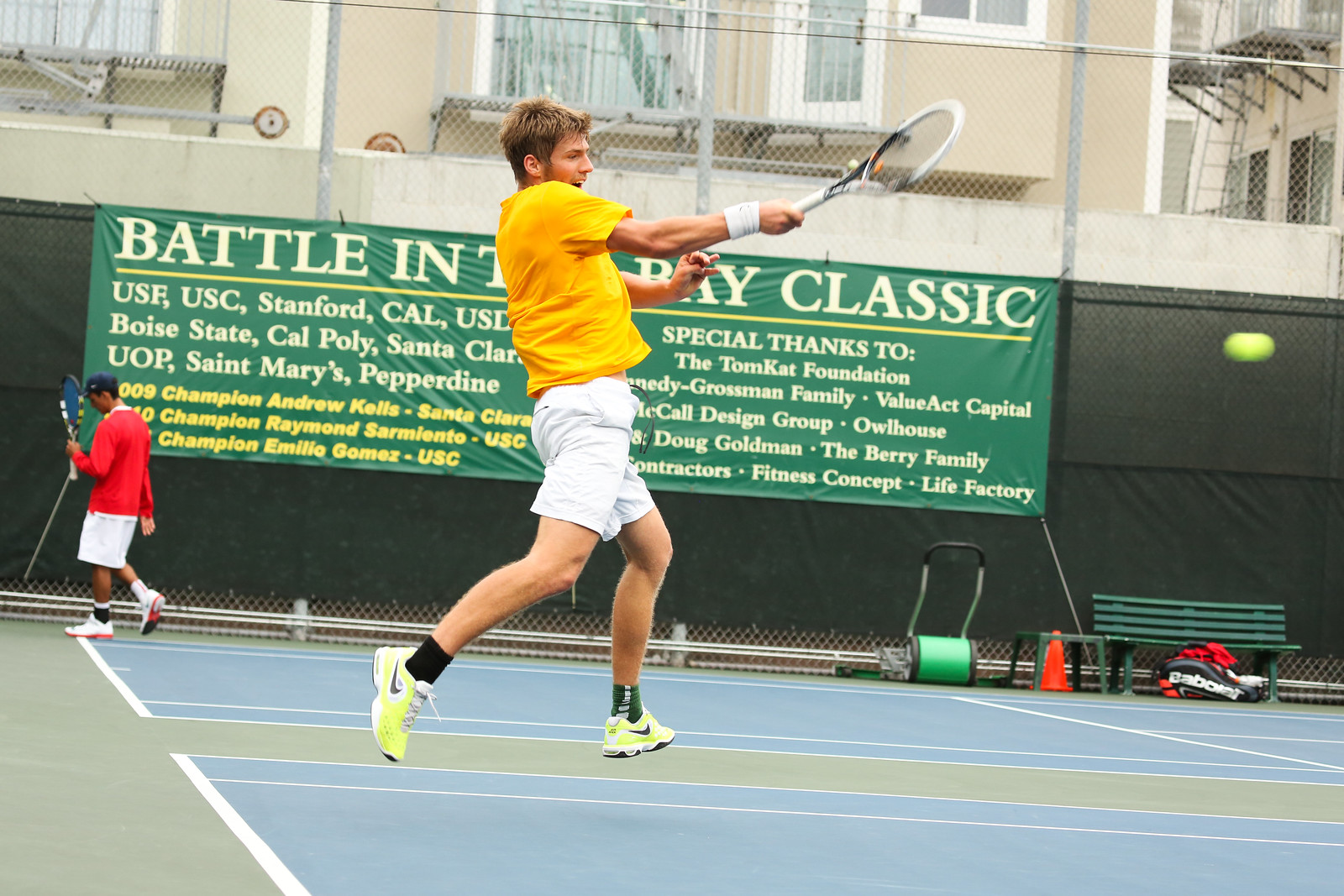The photograph captures a young, light-skinned male tennis player in mid-air, caught perfectly in mid-swing with a white and black tennis racket. His attire includes a yellow jersey, white shorts, white and green Nike tennis shoes, and a white wristband on his right wrist. The tennis ball he presumably just hit is visible in the distance to the right side of the image. The brightly lit scene is set on a blue tennis court surrounded by green areas, with multiple courts visible. In the background, a large green sign prominently displays "Battle in the Bay Classic" along with college names such as USF, USC, Stanford, and CAL, and acknowledges the Tomcat Foundation. Another tennis player, donning a red shirt, white shorts, white shoes, and a black hat, appears to be walking away at the edge of the court. The setting includes high chain-link fences and distant buildings, all illuminated by natural light, emphasizing the clear and vibrant atmosphere of the event.